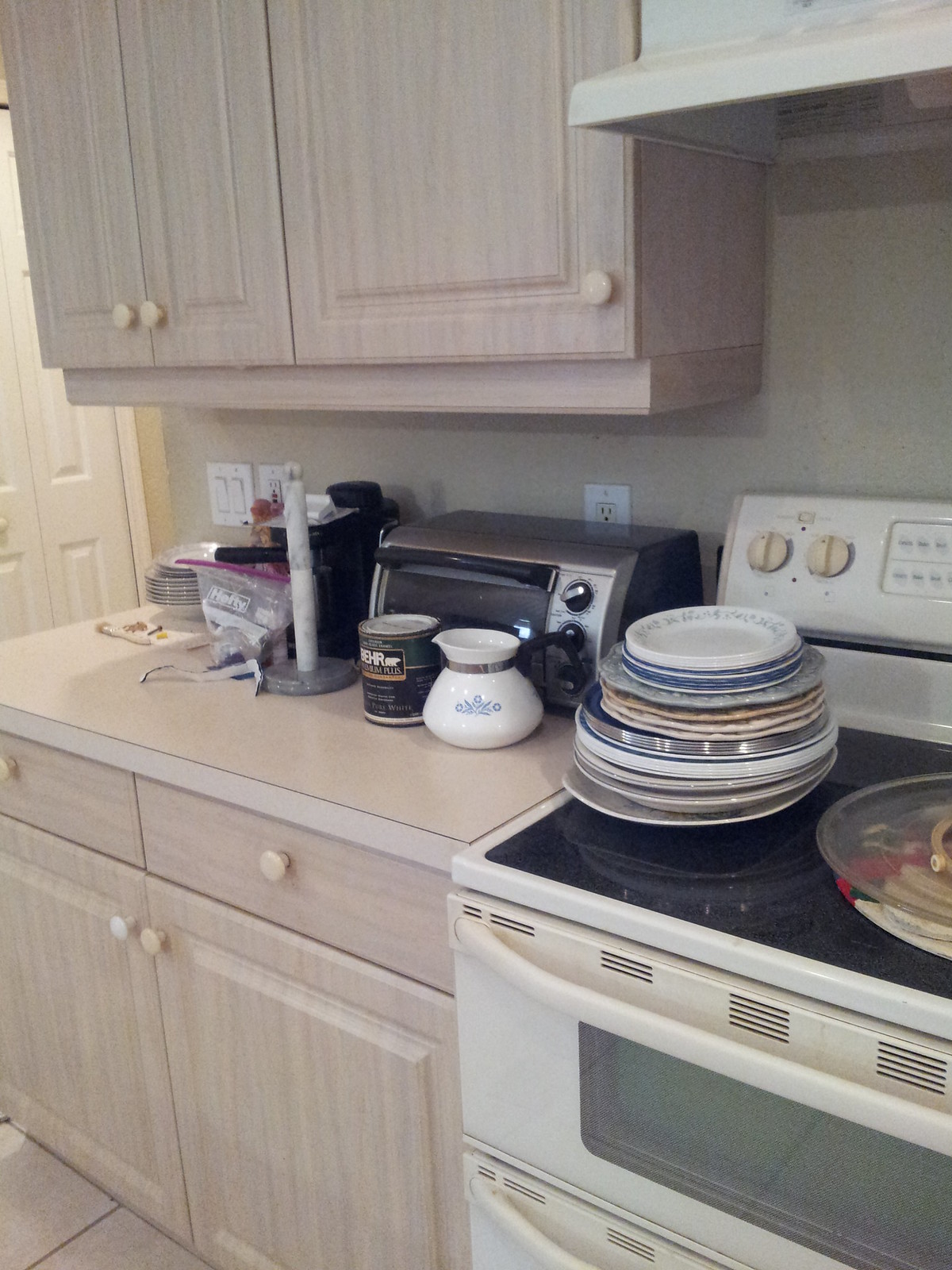The image showcases a well-organized kitchen with a blend of neutral tones and modern design elements. The kitchen features very pale, grayish-brown wooden cabinets with a raised panel design. Each cabinet is adorned with round beige-colored pull knobs. 

On the far left, there is a prominent white door with inset panels, revealing a small section of the wall outside the door. Mounted above the counter are three cupboards: the first two open outwards with center pull doors, while the third swings to the left. 

In the upper right-hand corner, a sleek stove hood is visible above a beige wall, which includes a white electrical outlet and a double light switch. Below the hood is a modern white flat-top stove with a black top. Two knobs are positioned on the left side of the stove, accompanied by push buttons. The stove's front left burner holds a stack of plates and paper plates in varying sizes and colors—white, blue, and brown with silver edges. On the front right burner, a potholder and a lid are placed.

Adjacent to the stove, a light beige countertop extends leftward. Positioned against the back wall is a black toaster oven with a chrome front, revealing its interior. Beside the toaster oven is a white corningware coffee pot with a cornflower design. A metal can labeled "BEHR" is situated next to the coffee pot. Further along the counter, near the door, stands a paper towel holder with a gray base, accompanied by a black sack and a Ziploc sack. Underneath the light switch, another stack of bowls is neatly arranged.

Below the countertop is a set of cabinetry: two drawers with round pull knobs and two cabinets that open towards the center. The stove also includes an additional drawer or potentially a secondary oven for extra storage or cooking capacity. The entire kitchen exudes a harmonious, neutral color palette with efficient storage and functionality.